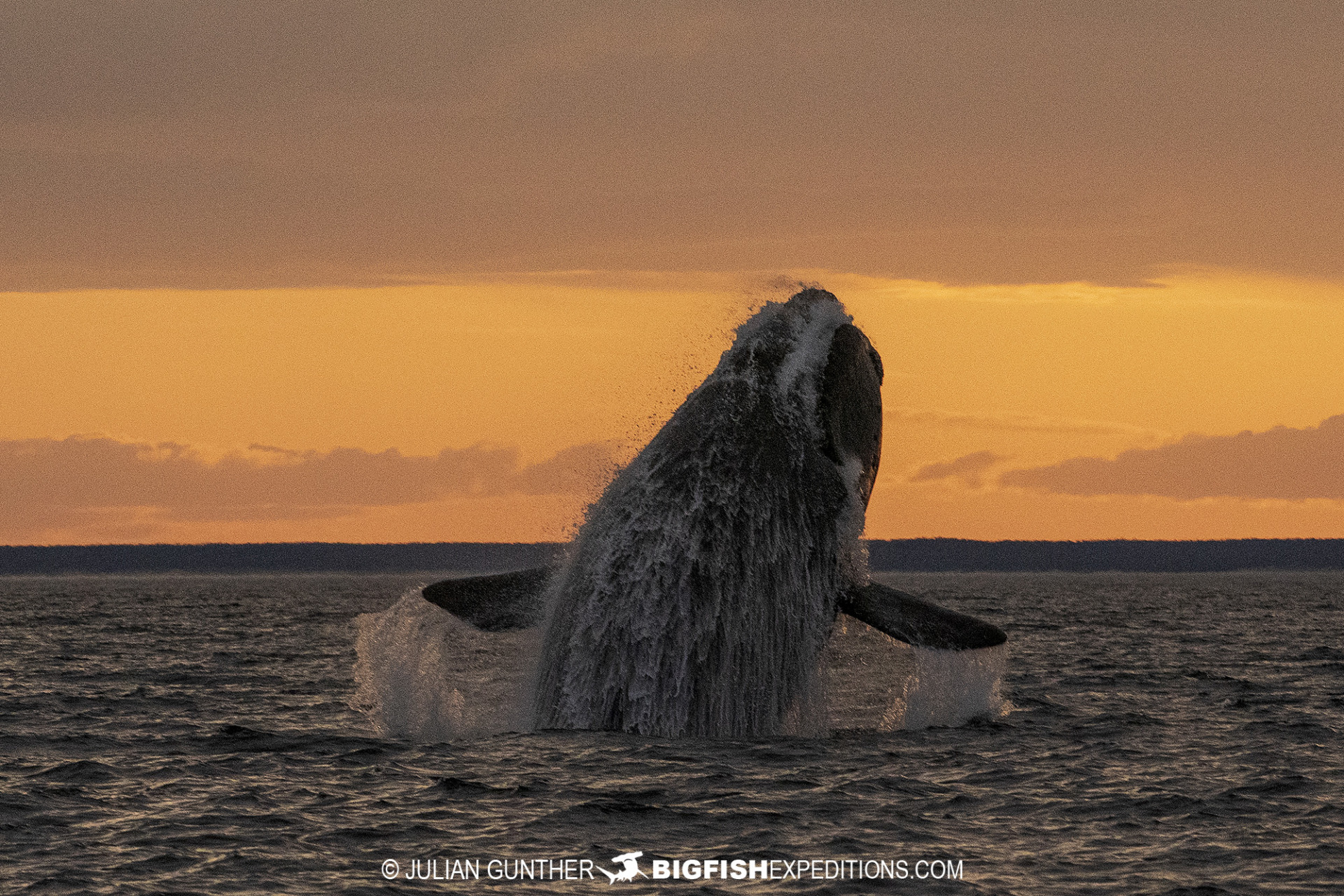In this striking photograph by Julian Gunther (bigfishexpeditions.com), an orca whale dramatically breaches the ocean surface, with water cascading off its body and fins, creating a spectacular splash. The choppy waves reflect an intense orange and yellow sunset sky, contrasted by scattered dark and grayish-orange clouds. Far off in the distance, a faint shoreline marks the horizon. The rich colors of the sunset bathe the scene in a warm, glowing light, emphasizing the dynamic motion and majesty of the whale. The copyright notice "Julian Gunther" and the logo featuring the text "bigfishexpeditions.com" with a bold white "BIGFISH" and a hammerhead shark silhouette are prominently displayed at the bottom of the image.